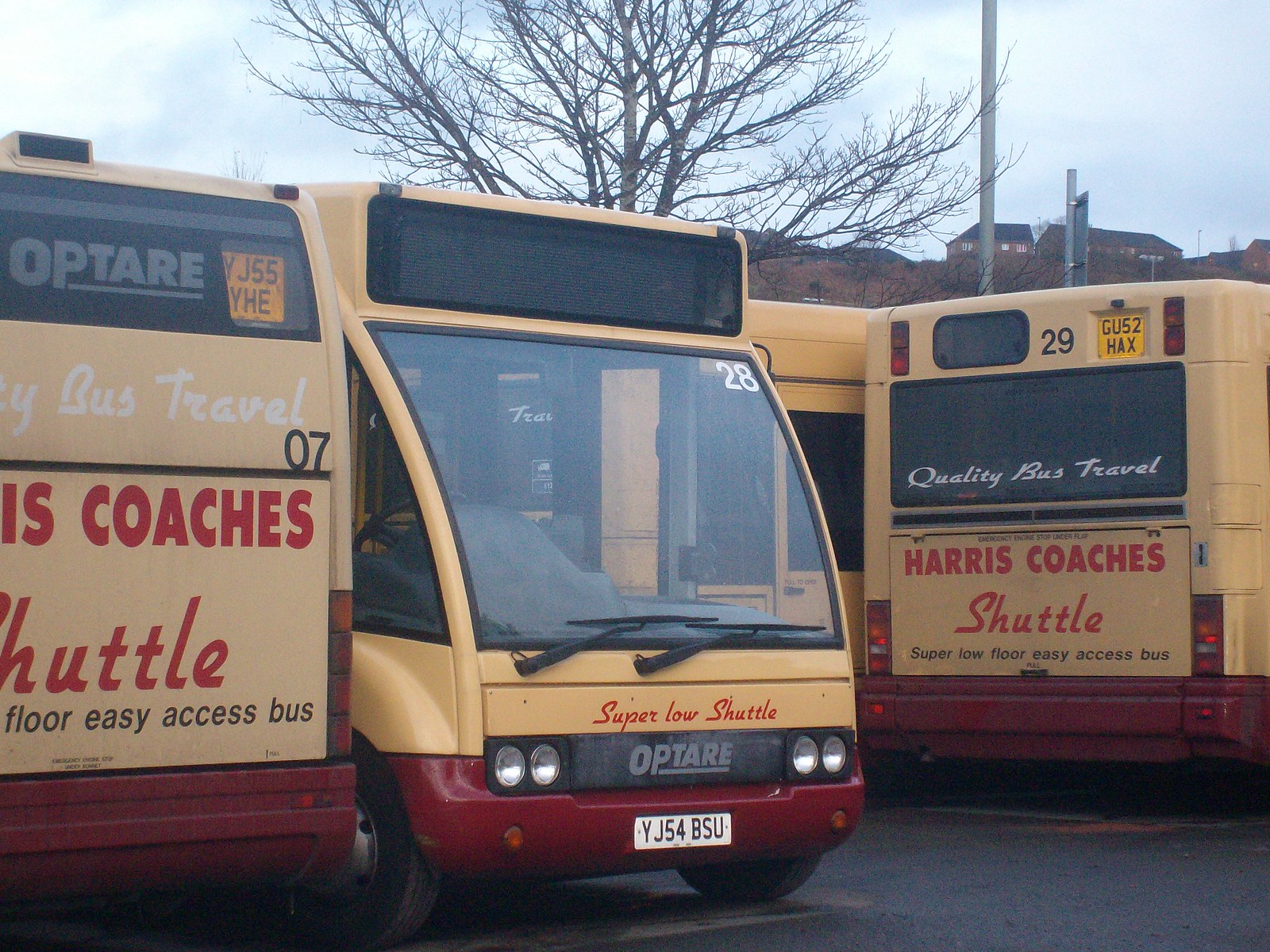The image depicts a busy shuttle bus parking area, featuring several buses that appear to be non-American, likely from England. The prominently visible buses are red and yellow-tan with large front windows. Each bus is labeled with "Harris Coaches Shuttle" and promotes "super low floor easy access bus" for quality travel. Buses are numbered 7, 28, and 29. They are parked in diverse orientations—some pulled in straight, others reversed into their spots. License plates like "GU 52 HAX" suggest a non-American origin. In the background, a hill slopes upwards adorned with buildings, while a tree provides some natural scenery. The setting is a spacious parking lot filled with multiple shuttles, indicating a transit or bus depot.